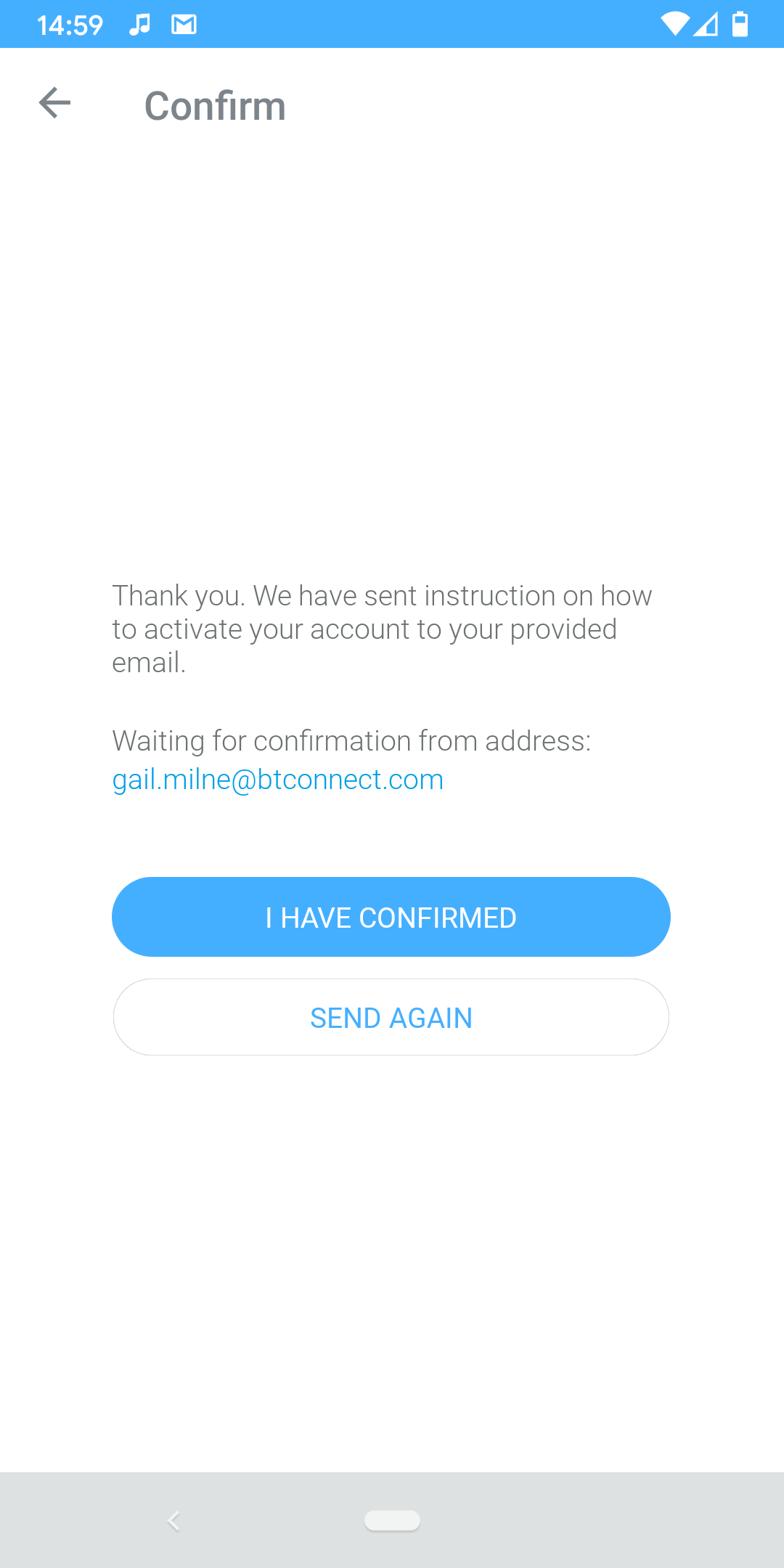The image portrays a digital confirmation screen with a structured layout and various icons and messages.

At the very top, within a blue banner, the time "14:59" is displayed in white text. To the right of the time, there is a musical note icon followed by another unspecified icon. Further to the right, there is a battery meter, a Wi-Fi symbol, and a white funnel icon.

Below this banner, a left-pointing arrow is accompanied by the word "Confirm." The central part of the screen contains a message that reads: "Thank you. We have sent instructions on how to activate your account to the provided email." 

Directly beneath this message, it states: "Waiting for confirmation from address gal.ml.milany@btconnect.com."

Further down, a blue button displays the text "I have confirmed," and below that, a white button with blue text reads "Send again."

At the bottommost part of the screen, a long gray block spans the width, with a small, faint white line running horizontally through its middle.